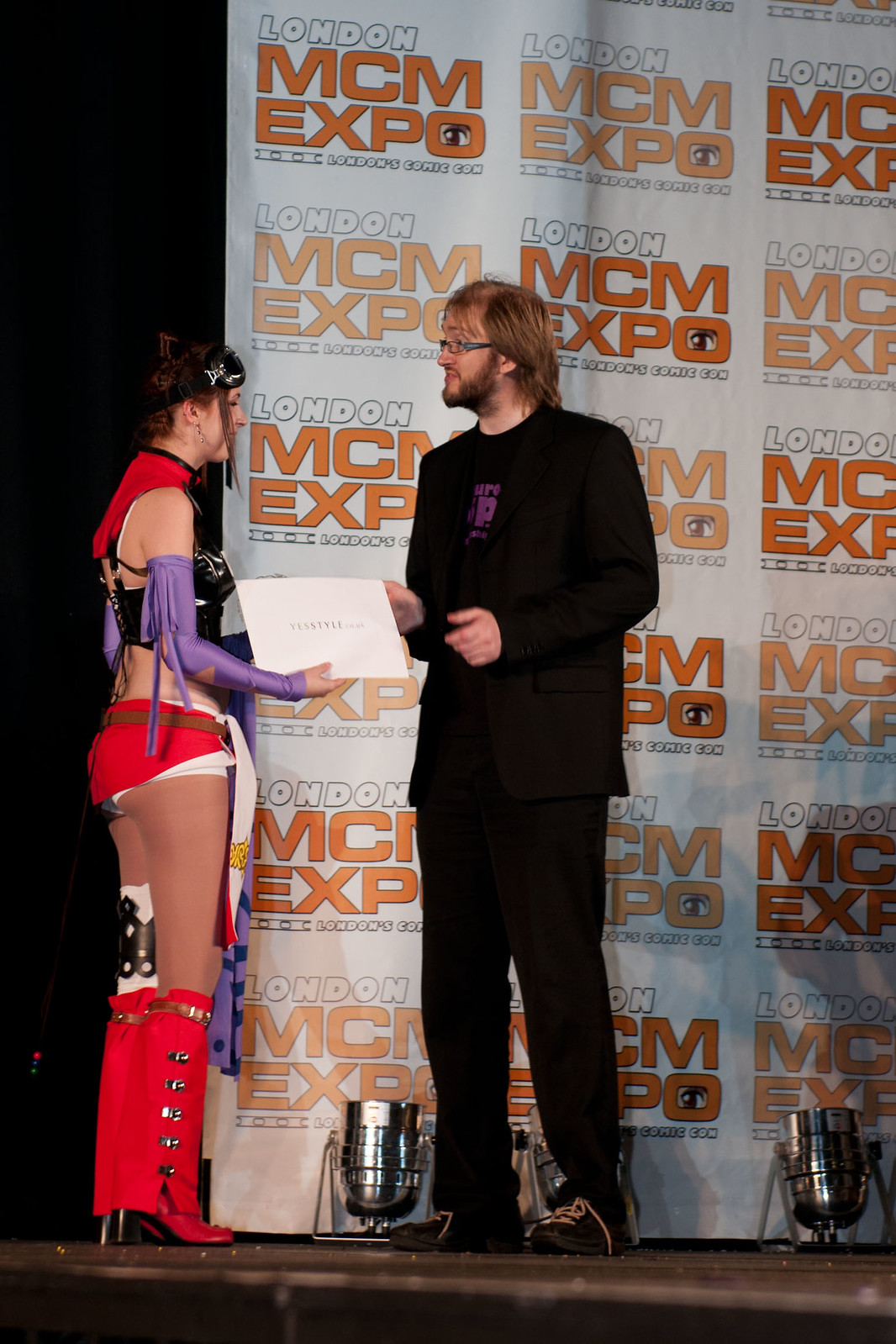In this photograph taken at the London MCM Expo, two individuals are captured on stage amidst a backdrop repetitively displaying "London MCM Expo". The woman, positioned to the left, is cosplaying a video game character with a vibrant outfit that includes a red top with bare shoulders, purple sleeves, a black halter top, pink shorts, and reddish-pink boots, leaving her midriff and upper thighs bare. She is holding out her hand and appears to be saying something to the man on her right. The man, who stands centrally in the frame, has reddish-brown hair, glasses, and a beard. He is dressed in a black suit with an open jacket revealing a black t-shirt with an emblem obscured by the coat, and paired with dark sneakers. He is in the process of presenting her with an award, and both subjects appear happy. Stage lights installed below illuminate the area while the large curtain behind them clearly states "London MCM Expo," with an anime-style eye embedded in the letter "O," emphasizing the event's connection to London's Comic Con.